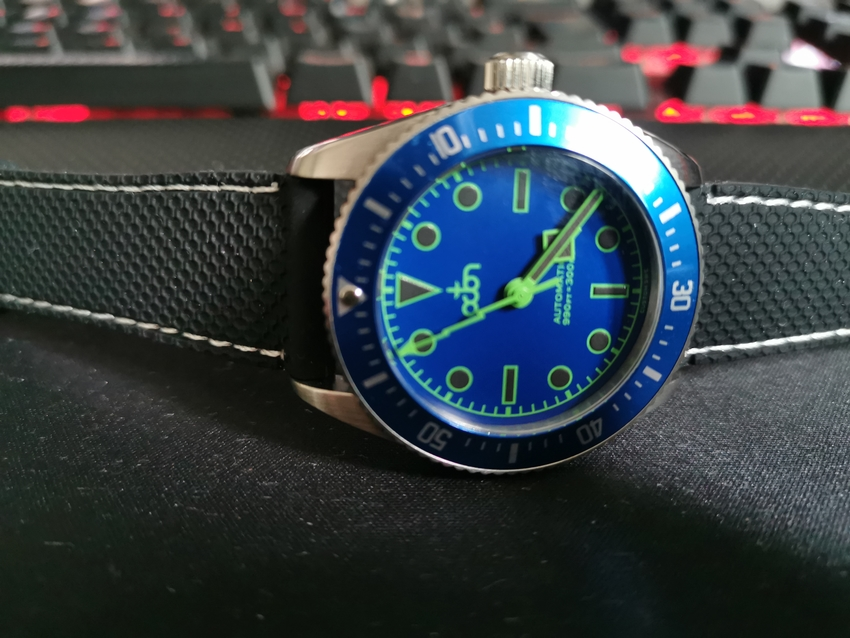The photo depicts a vivid indoor scene, likely taken on a desk setup. Dominating the foreground is a blue wristwatch laid out across a dark surface that appears to be a mouse pad. Behind the watch, a blurred keyboard with a striking red glow under its keys suggests it is active, casting a subtle light over the scene. The keyboard is identified as a standard QWERTY type.

The wristwatch, which is the focal point of the image, features black cloth straps with white stitching along the edges. Metal clasps connect these straps to the metallic blue watch face, which is encircled by a silver bezel. The watch face itself is a deep blue, featuring contrasting white numerals around the outer edge and unique green-outlined shapes—circles, squares, rectangles, and triangles—marking the hours. The clock hands, finished in green, complement the overall color scheme. Numerals such as 50, 40, 30, 20, and 10 are visibly inscribed around the watch face, adding to its detailed design. This detailed snapshot is likely captured in a home or work environment, highlighting both function and style.